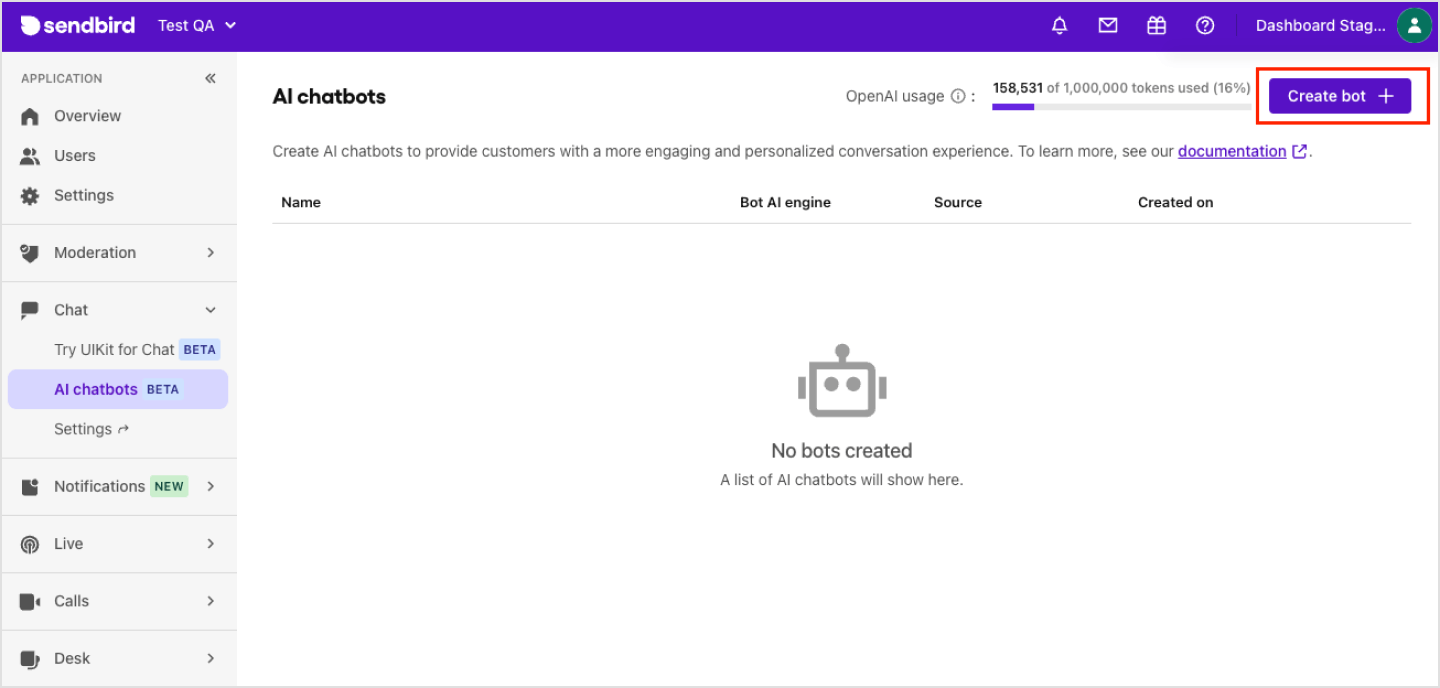The image depicts a user interface for Sendbird, predominantly featuring a white background with a distinctive purple-blue border at the top. The top section showcases the Sendbird logo followed by the text "Test QA." On the right side of the header, there's a row of icons: a bell (likely an alarm icon), an image icon, a gift-like icon, a question mark icon, and a user icon next to the text "Dashboard Staging" (or similar), presumably for account management.

The left side of the interface contains a light gray sidebar labeled "Application" at the top, with various categorized menu items: 
- "Overview" with a Home icon
- "Users" with a People icon
- "Settings" with a Gear or Cog icon
- "Moderation"
- "Chat," which includes options for "Try Chat Beta," "All Chatbots Beta Settings," 
- "Notifications" (marked as new)
- "Live"
- "Calls"
- "Desk," each accompanied by relevant black icons.

Central to the main screen is an "AI Chatbots" section, displaying "Open AI Usage" with a status of "150,000 out of 1 million tokens used" (16% in parentheses). Below this, there is a red-outlined rectangle with the same purple-blue hue saying "Create Bot Plus," which users can click on to create a chatbot. The section explains the purpose of AI chatbots for delivering a more engaging and personalized conversation experience, with a hyperlink to the documentation for further information.

The main content area lists four columns: "Name," "Bot," "AI Engine," "Source," and "Created On." A vintage robot head icon is shown with the message "No Bots Created," indicating that this is where the list of AI chatbots would appear once created.